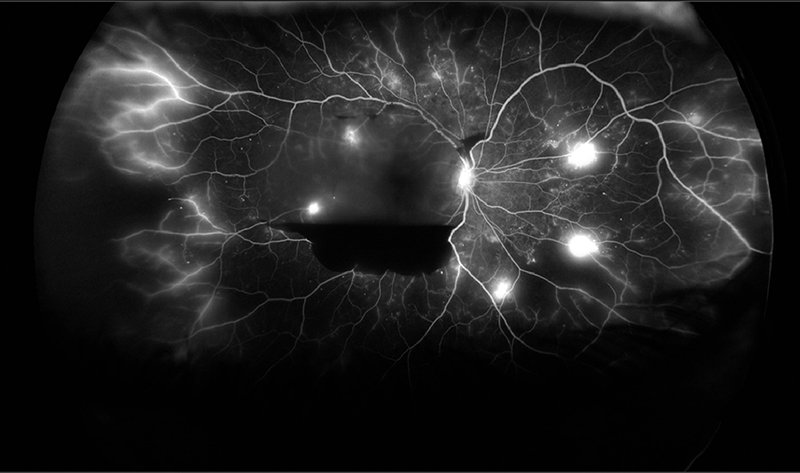This image appears to be an x-ray, predominantly in black and white, with no identifying text or context. It features a central, oblong, and possibly circular formation that is filled with intricate, vein-like or nerve-like patterns. Scattered throughout this shape are approximately five small, bright white spots, concentrated mainly in the center, accompanied by a few smaller white dots along the edges. Surrounding these central spots, the white bursts create a lightning or plasma-like appearance, with cracks and fractal patterns extending outward. The background of the image is solid black, and the object itself has a dark gray hue, giving it a cloudy texture with flashes of light. This formation vaguely resembles a crystal ball or an abstract eye, with the bright veiny structures radiating throughout the image.